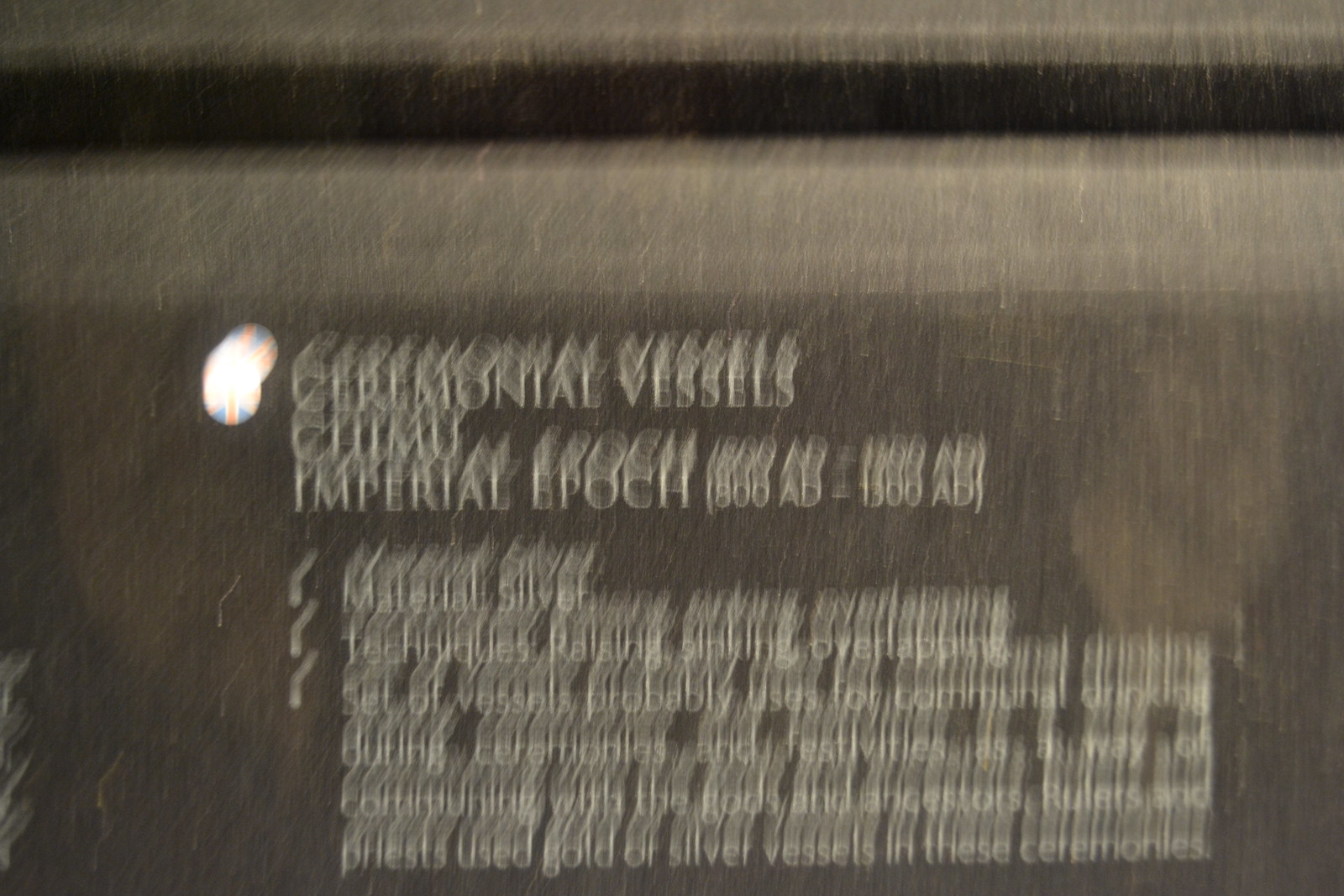This photograph captures a very blurry image of what appears to be a decorative stone placard, featuring lighter-colored stone at the top and dark gray or brownish hues. Despite the lack of clarity, white text on the upper middle portion of the placard can be discerned, detailing information about "Ceremonial Vessels" from the Chimu Imperial Epoch, circa 800 A.D. to 1300 A.D. Below this heading, bullet points list "Material: Silver" and various crafting techniques, including "Raising, Sinking, Overlapping." The text suggests that this set of vessels was probably used for ceremonial drinking during ceremonies and festivities, likely serving as a means of communicating with the gods and ancestors. Details also mention that rulers and priests used gold or silver vessels in these ceremonial contexts. The rest of the text is too blurry to read, and there is a small British flag depicted beside the ceremonial vessels.